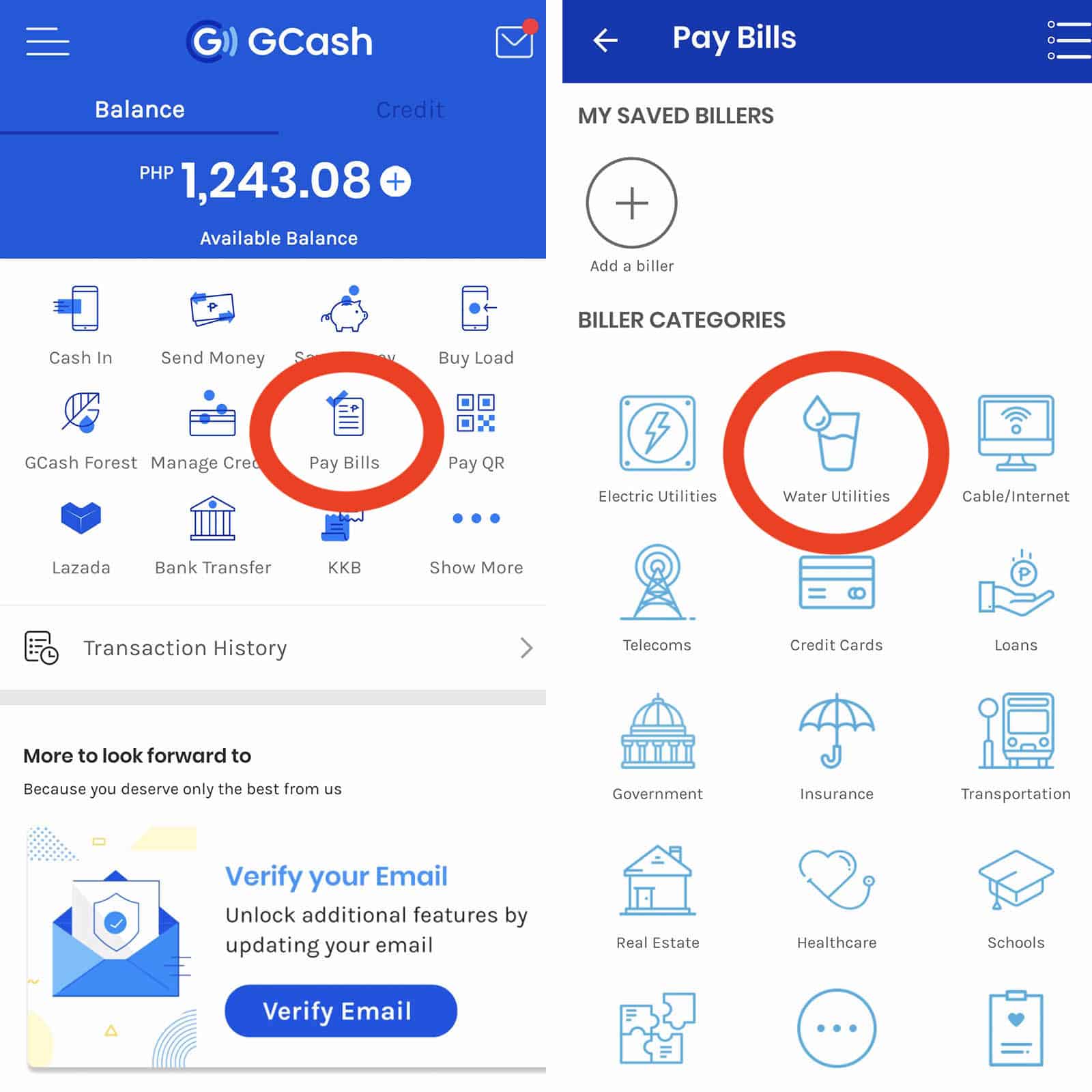This is an informative side-by-side photo displaying the interface of a financial application, specifically GCash. Each image is in portrait orientation with a thin white boundary separating them. 

The first image features the main screen of the GCash app. At the top, there is a blue rectangular bar with the GCash logo and name prominently displayed. To the upper right, a small envelope icon with a red notification dot suggests the presence of an unread message. Below this, there are two tabs labeled 'Balance' and 'Credit', with 'Balance' highlighted, showing an available balance of PHP 1,243.08. Several options are visible within the app, such as 'Cash In', 'Send Money', among others, with 'Pay Bills' selected and highlighted with a red circle.

The second image focuses on the 'Pay Bills' section of the GCash app. It has a smaller blue bar at the top, featuring the 'Pay Bills' title in white text, a back arrow icon on the left, and a hamburger menu icon on the right. The majority of the screen has a white background. Below the title bar, 'My Saved Billers' is listed, with an option to add a new biller. Further down, under 'Biller Categories', several options are available, including 'Electric Utilities', 'Water Utilities', 'Cable Internet', 'Telecoms', and 'Credit Cards'. The 'Water Utilities' category is selected and circled in red, indicating the demonstration focuses on how to pay a water utility bill via the app.

The image as a whole seems to serve as a detailed guide on navigating the GCash app's bill payment features, particularly for paying water utility bills.